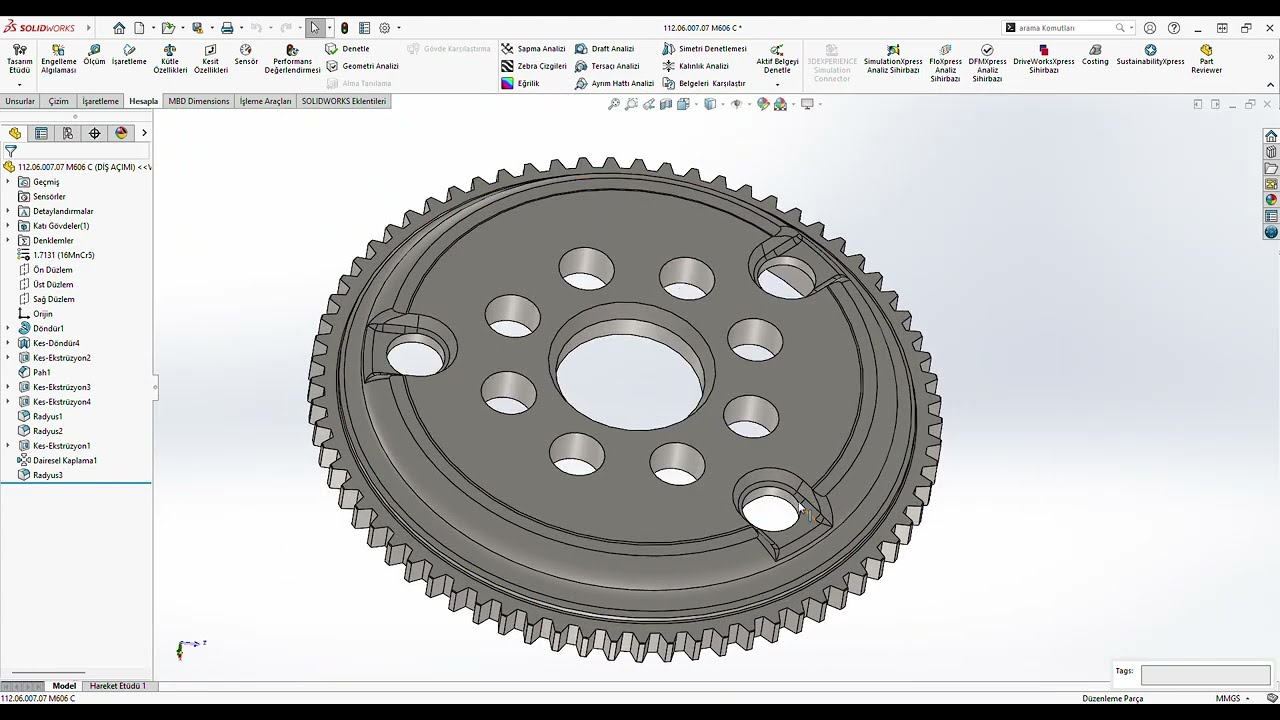This image is a detailed screenshot of a computer-aided design (CAD) software, identified as SolidWorks, opened on a computer screen. The right-hand section prominently features a 3D graphical representation of a metal gear on a grey background with a gradient effect. The gear has fine, symmetrical teeth along its edge. At the center of the gear, there is a large circular hole surrounded by several smaller holes, while the outer edges feature three evenly spaced circular holes.

The software's interface includes a top menu bar with icons and typical webpage symbols such as a home button, print option, navigation arrows, search bar, and a button to resize the window. The left-hand side has a side menu with various options, potentially for layers, motions, or drawing tools. Some of the text appears to be in a foreign language, indicating that this version of SolidWorks may be tailored for an international audience.